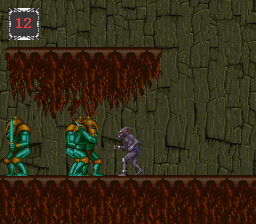In what appears to be a vibrant video game scene, four distinct characters are positioned against the backdrop of a towering gray rock face. Emerging from the rock face are curious red coiled structures, possibly representing plants, adding a mystifying element to the environment. The characters stand on a flat plateau, beneath which more of these coiled red strands of matter can be seen, enhancing the surreal atmosphere. Three of the characters are clad in matching turquoise suits, accented with gold plates on their knees and shoulders, and they wear gleaming gold helmets. The fourth character contrasts sharply with the others; it is a small, purple, alien-like creature adorned merely in a blue loincloth, its body otherwise naked. This creature features a pointed head and an alien visage, adding a further layer of intrigue to the scene.